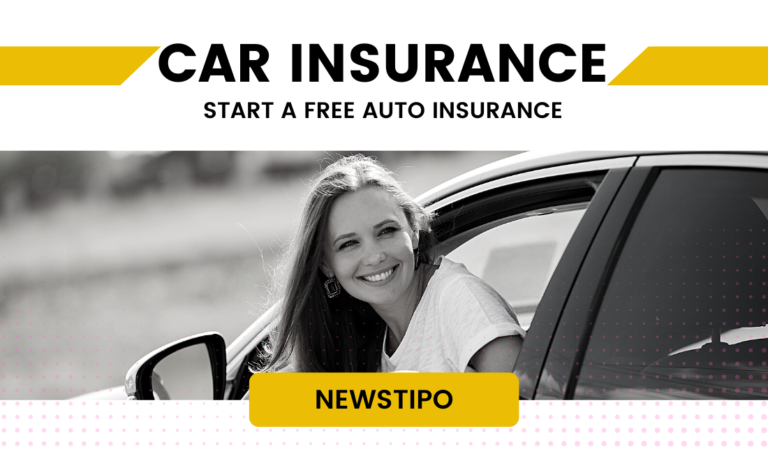The image is an advertisement for car insurance with a predominantly white background. The center to bottom two-thirds of the image features a horizontal, black-and-white photograph. Across the top of the image, there is a partially visible yellow banner, intersected by a section with white background and black, bold, capitalized text that reads "CAR INSURANCE." Beneath this, the white background continues with smaller, black, capitalized text that states, "START A FREE AUTO INSURANCE."

At the very bottom center of the image, there is a yellow rectangle containing the text "NEUSTIPO" in black, capital letters. The bottom portion of the photo incorporates a faint grid dot pattern with light pink dots, subtly fading towards the center of the photograph. The black-and-white photo itself captures a young woman with long dark hair, smiling as she leans out from the driver’s side window of a car. She is wearing a white, short-sleeved t-shirt.